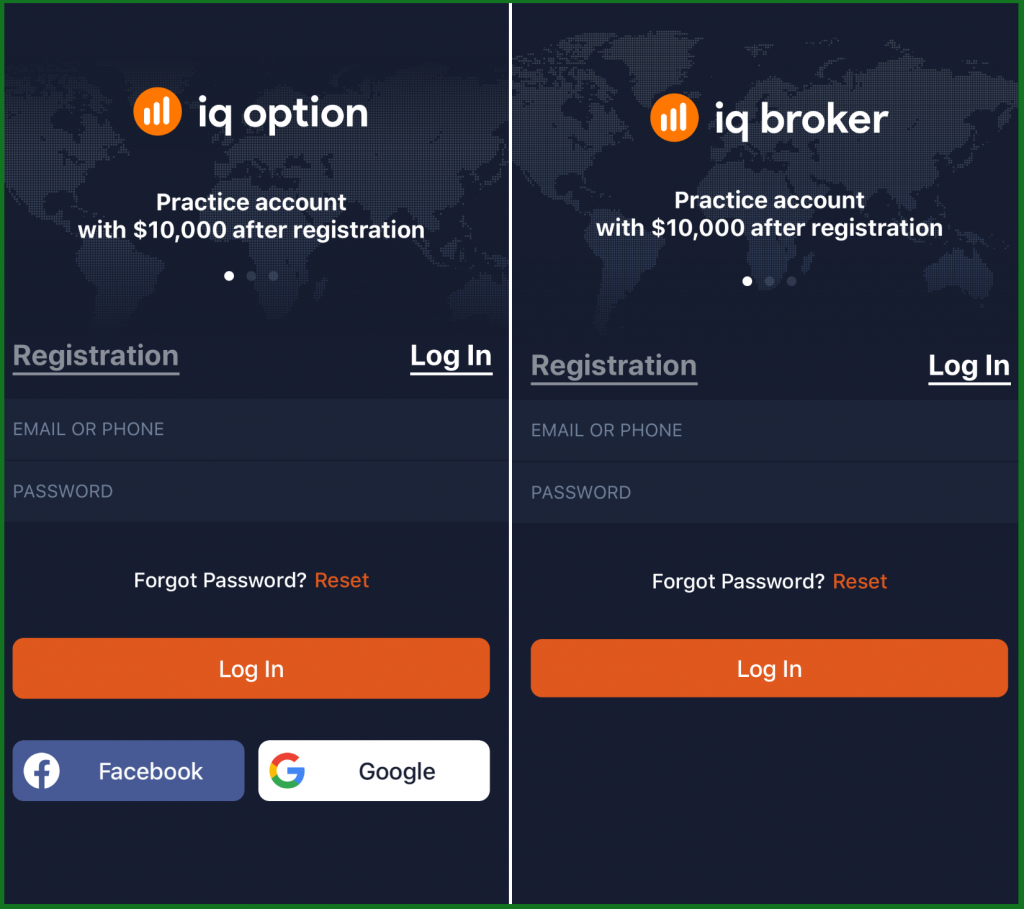The image consists of two nearly identical screenshots placed side by side in two columns, likely taken in portrait mode from a cellphone. Each screenshot features the interface of the IQ Option app displaying a practice account with a $10,000 balance after registration. The top section of both screenshots features the label "IQ Option" and "Practice Account," followed by text indicating the user is on the first tab.

Below this, there is a "Registration Login" section that is highlighted, with input fields for "Email or Phone" and "Password" written in light gray. Beneath these fields, the prompts "Forget Password" and "Reset" appear. 

The significant difference between the two screenshots lies in the login options: the left screenshot includes the option to log in via Facebook or Google with corresponding buttons, while the right screenshot does not feature these social login options. Both screenshots have a large "Login" button under the "Forget Password" and "Reset" prompts.

The upper portions of both screenshots display a dark background featuring a world map in shades of dark gray and black, while the rest of the interface maintains a predominantly black background. This subtle difference in the availability of social media login options seems to be the primary focus of what is being displayed.